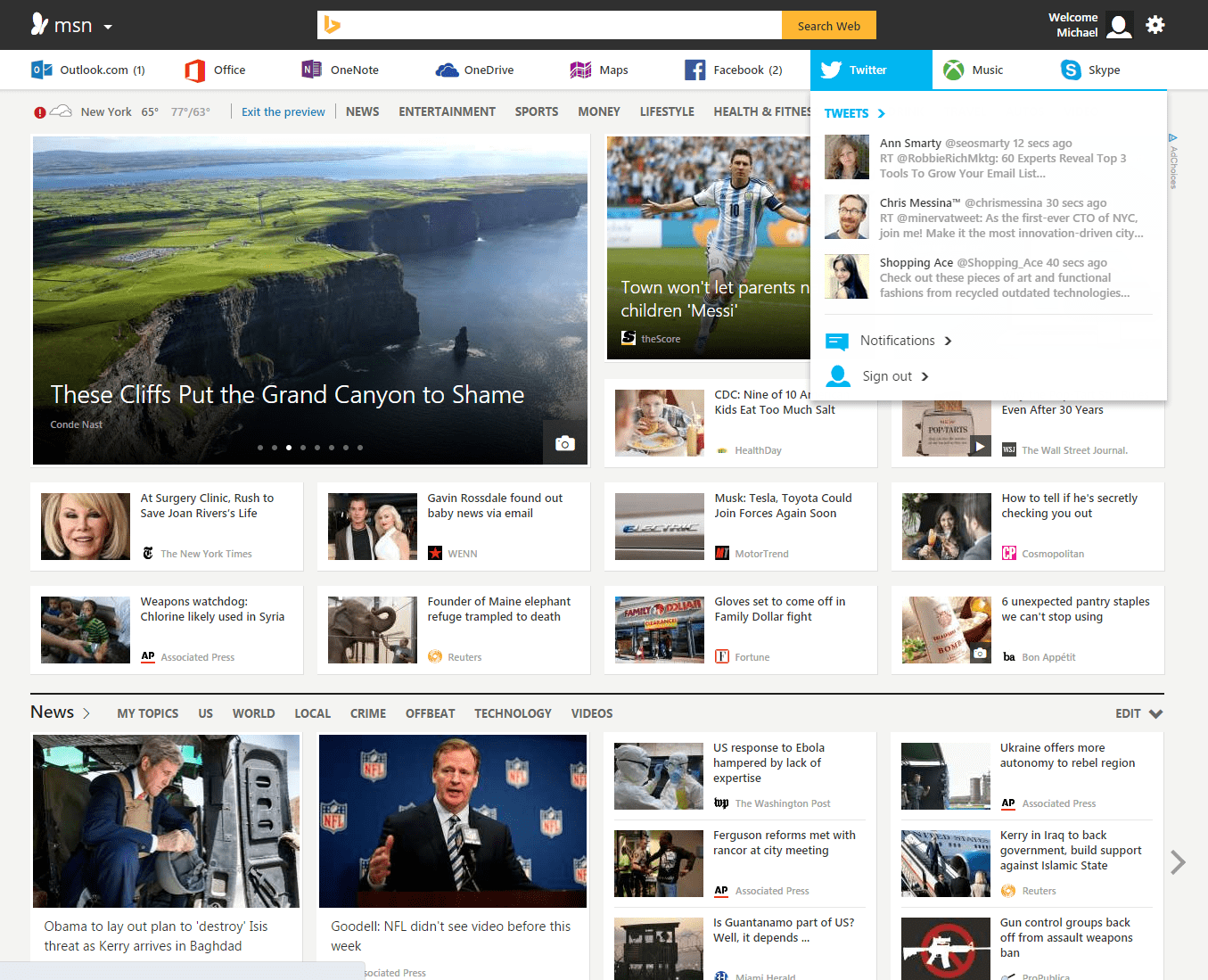A screenshot of an MSN website is displayed, featuring a sleek, dark gray-black header adorned with a butterfly logo next to the text "MSN" and a downward-pointing arrow. Centrally positioned beneath the header is the Bing search bar, accompanied by a yellow “search web” button. 

At the top right corner, a welcoming message reads "Welcome Michael," alongside an icon depicting a simplistic white circle resembling a face and body. The top navigation menu offers various Microsoft services and social media options: Outlook.com, Office, OneNote, OneDrive, Maps, Facebook, Twitter, Music, and Skype, with Twitter actively selected and showcasing a few tweets. Options to view notifications or sign out are also present.

Below the social media integration, the main content is dominated by several news articles. To the left, the most prominent headline reads, "These cliffs put the Grand Canyon to shame," accompanied by an image of stunning cliffs and water. Adjacent is a photo of a soccer player, followed by numerous additional headlines with smaller images, including:

- "At surgery clinic, rushed to save Joan Rivers' life."
- "Weapons watchdog: chlorine likely used in Syria."
- "Gavin Rossdale found out baby news via email."
- "Founder of Maine elephant refugee trampled to death."
- "CDC: 9 of 10 kids eat too much salt."
- "Muck Tesla, Toyota could join forces again soon."
- "Gloves said to come off in family dollar fight."

A myriad of other headlines and stories continue below, providing a comprehensive snapshot of diverse news topics and updates.